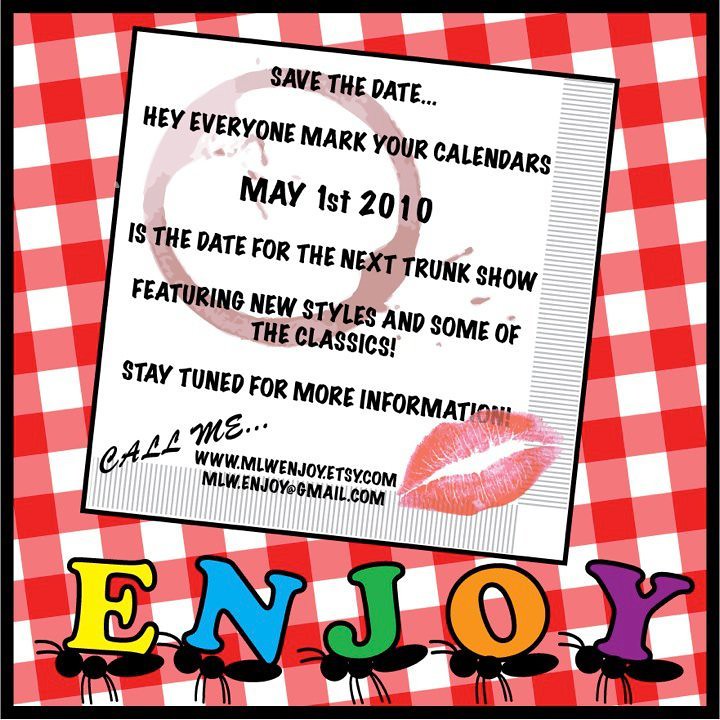This advertisement for a trunk show features a background resembling a red-and-white checkered picnic cloth, bordered by a thin black line. At the top, a slightly tilted grey square with a coffee and lipstick stain serves as a focal point, bearing the event details in black font. It reads: "Save the Date. Hey everyone, mark your calendars. May 1st, 2010 is the date for the next Trunk Show featuring new styles and some of the classics. Stay tuned for more information. Call me, www.mlwenjoy.etsy.com, mlw.enjoy@gmail.com." Below this text, five cartoon ants march across the ad's bottom, each carrying a colorful letter that together spell "ENJOY" in yellow, blue, green, orange, and purple.